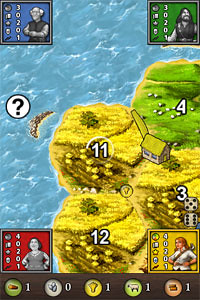This detailed caption provides an in-depth description of the screenshot:

"A captivating screenshot from a mobile video game, showcasing its interface. The bottom of the screen features five distinct icons representing different resources: a green icon with wood, followed by stone, wheat, sheep, and brick. The map displayed in the screenshot is divided into four sections, with a notable landmass area and a blue and white water region. In the upper right corner of the green section is the number '4', while the three yellow sections are marked with '11', '3', and '12' respectively, each likely indicating resource quantities or points.

At the center, a white circle with a black question mark provides navigational or help options. Additionally, four character avatars occupy the corners of the screen: the upper left corner features an older man in blue, the upper right corner shows a younger man with long hair in green, the bottom left presents a woman in black and white on a red background, and the bottom right displays a woman with red hair in a white shirt, bordered with yellow. This screenshot effectively captures the essence and intricate layout of the game."